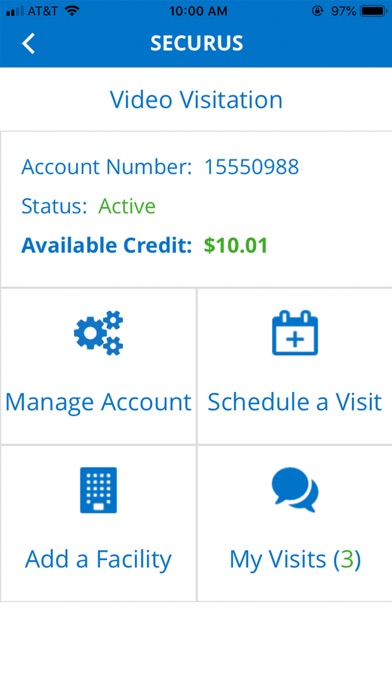In this image, we observe a screenshot of a mobile device's interface. On the top-left corner, the network signal indicator displays 2 out of 4 bars, with the service provider listed as AT&T. Centrally positioned at the top of the screen, the time is displayed as 10:00 AM. Additionally, the screen orientation is locked, as indicated by the lock icon. On the top-right corner, the battery level shows a robust charge of 97%.